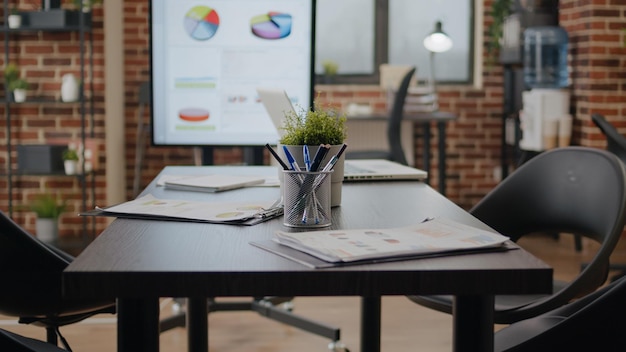The photograph portrays a small conference room within a small business office. The focal point is a modern black table flanked by two matching black chairs. On the table, there is an arrangement that includes a mesh container filled with pens, an open laptop, a tablet, and two white notebooks or periodicals. Also on the table is a small plant pot with greenery, adding a touch of nature to the setting. 

In the background on the right side, an exposed red and brown brick wall adds a rustic touch to the office environment. A water cooler with a dispenser and cup holder stands in the back right corner. Beside it, a table with an illuminated gooseneck lamp and some books creates a cozy scene. Central to this backdrop is a screen displaying various pie charts and graphs, indicative of a business meeting or presentation. To the left of the screen, a black iron shelving unit adorned with plants, vases, and knickknacks adds decorative and practical elements to the space. The overall atmosphere is a blend of modern functionality and homely decor, creating a welcoming yet professional environment.